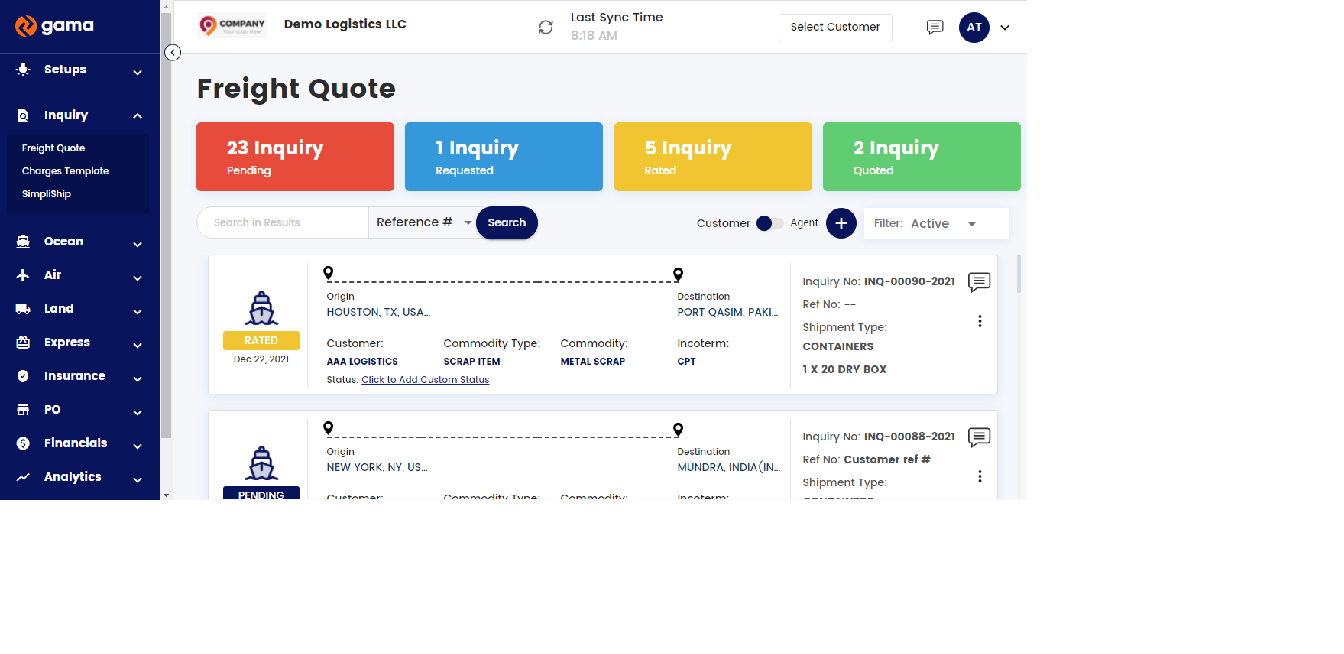The image displays the user interface of a site named Gamma, prominently featuring its logo and name in the top-left corner. Opposite this, a white panel provides details about a company, specifically Demo Logistics LLC. Centrally, there's a sync button and the last sync time displayed, with an option to select a customer. A drop-down menu labeled "AT" indicates options for the logged-in user.

On the left-hand side, a dark blue panel lists various selectable options including Setups, Inquiry, Ocean, Air, Land, Express, Insurance, PO, Financials, and Analytics, pointing towards a freight company’s operations. The main panel in the center focuses on freight inquiries, highlighting the selection under "Inquiry". It shows four colored rectangular indicators of inquiries: orange (23 inquiries), blue (1 inquiry), yellow (5 inquiries), and green (2 inquiries).

Beneath these rectangles, detailed information about shipments is provided. This includes icons representing a ship, origin and destination locations, customer details, commodity type, final port of destination, and the number of containers onboard.